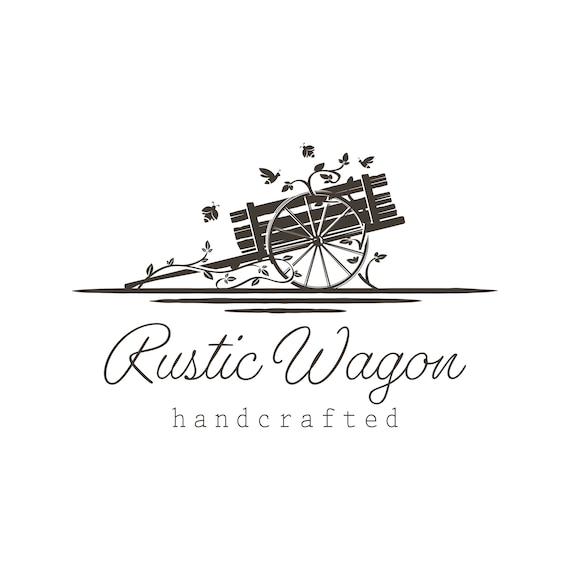This is a hand-drawn or computer-generated logo for a company called Rustic Wagon. The illustration, set against a white background, features a detailed depiction of an old wooden cart. The cart, which looks like it could be hand-pulled or drawn by a donkey, has a large wagon wheel and wooden planks forming its back. The handle is leaning against the ground on the left side, wrapped in small vines with petite leaves that also wind through the wheel. Around the top of the cart, various insects, including bees and other pollinators, are in flight. The cart rests on a trio of horizontal lines that decrease in size from top to bottom, providing depth and texture to the grounding. Below the image, "Rustic Wagon" is written in a script font, followed by the word "handcrafted" in a rounded lowercase type. The logo's color scheme is limited to a dark, almost black shade, adding to its rustic and handcrafted appeal.